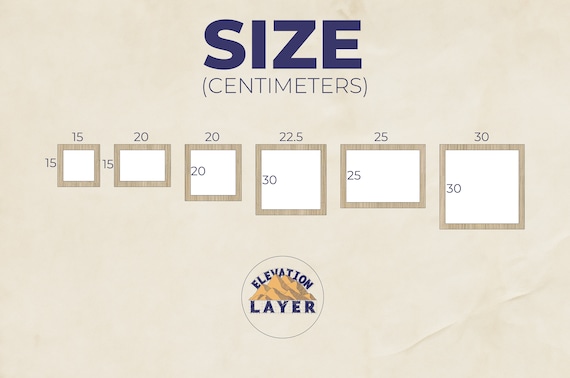The image, which has a landscape orientation, features an aged paper-like cream background. Across the top in large, bold, dark blue lettering is the word "SIZE," and beneath it, in smaller, all-cap letters within parentheses, is "CENTIMETERS." Central to the image are six square boxes arranged in a row, each delineated by brown borders with white centers and labeled with dimensions in navy blue text on the top and left sides.

From left to right, the first box is labeled "15" on both the top and the left side. The second box displays "20" on the top and "15" on the left. The third box has "20" both on the top and the left side. The fourth box, located centrally, shows "22.5" on the top and "30" on the left side. The fifth box features "25" on the top and the left side, and the final box has "30" labeled on the top and the left side.

Directly beneath these boxes, at the bottom center of the image, is a logo encased in a gray ring. This logo consists of the word "ELEVATION" curved above a depiction of mountain ranges, with the word "LAYER" in blue positioned below the mountains.